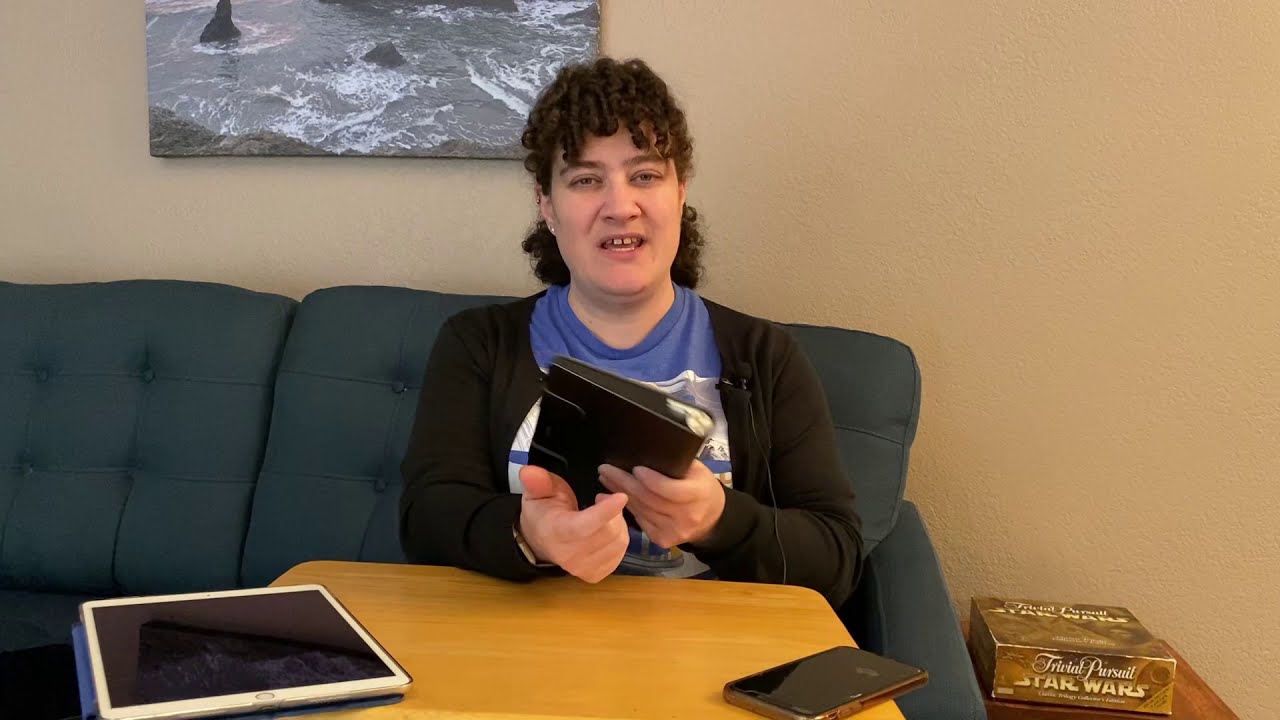In the image, a woman sits on a teal couch against a tan wall adorned with a black and white photograph of ocean waves crashing against rocks. She has medium-length, tightly curly black hair that falls just above her shoulders. The woman is clad in a blue t-shirt with a white logo, likely of a sports team, and a gray cardigan over it. She is engaged in conversation with the camera, appearing to describe or demonstrate the contents of a leather-bound case, which she is holding and pointing at. In front of her, a wooden TV tray serves as a workspace, featuring an iPad on the left and an iPhone on the right. To the left of the couch stands an end table with a Trivial Pursuit Star Wars edition box on it.